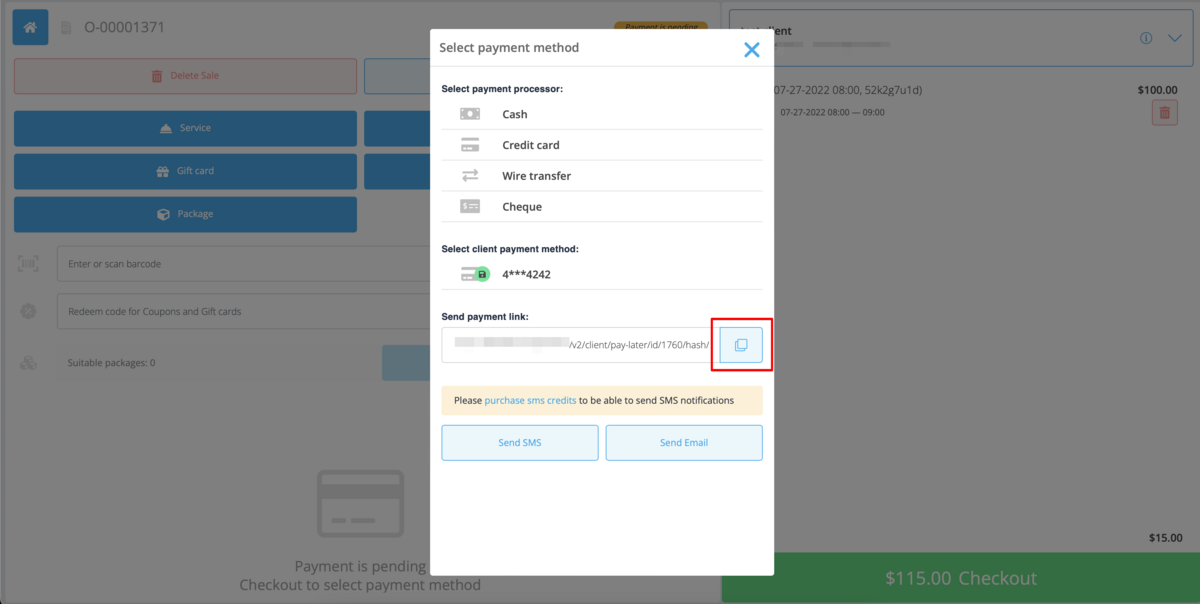A minimalist checkout page is displayed, indicating the purchase of an unidentified product priced at $115. The main page is grayed out, emphasizing a pop-up in the forefront dedicated to selecting a payment method. The user appears to have selected a debit card and entered their card number. There is an option to send a payment link, presented alongside an address field. This address is encapsulated in a highlighted box, designed for easy copying. At the bottom of the pop-up, options to send the payment link via SMS or email are available. Dominated by a green background, the page features predominantly white and blue elements, contributing to its clean and simple aesthetic.